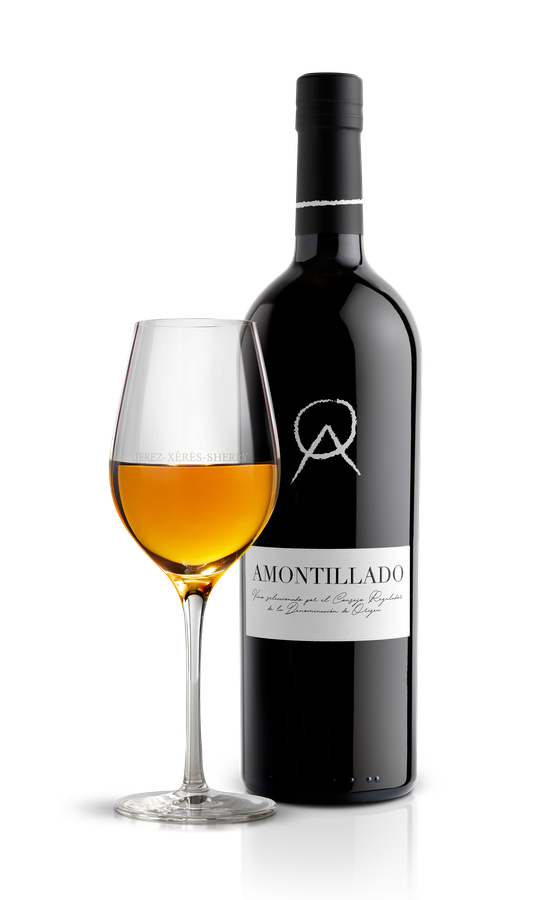The image features a black bottle of Amontillado prominently placed in the center against a white background. The bottle is capped and bears a circular and triangular logo in the middle of a white label, with the name "Amontillado" in black text, accompanied by smaller, harder-to-read cursive text beneath it. Next to the bottle, slightly overlapping its left side, is a half-full stemmed glass containing a golden or amber-colored liquid, suggesting the contents are a type of fortified wine rather than regular wine. The glass is designed with a round base and has a narrow, elongated bowl, indicative of flute-style drinkware. The composition is styled to emphasize the drinkware and the alcoholic product it holds.